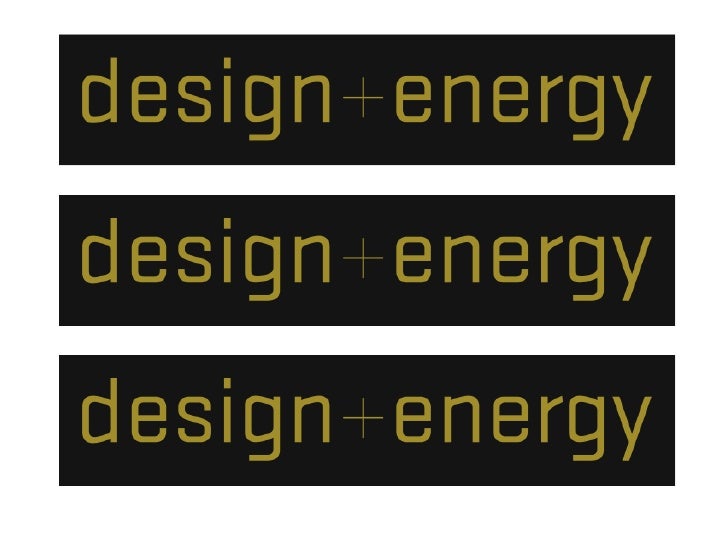The image displays three identical black rectangular signs, stacked vertically with a small white space between each one. Each sign, measuring approximately five times as long as they are tall, features the phrase "design plus energy" in a distinct, pea-greenish-yellow font. The text, including the tight plus sign between "design" and "energy," is perfectly aligned and repeated three times across the three signs. The overall arrangement and presentation emphasize the uniformity and repetition of the "design plus energy" message against the dark background.